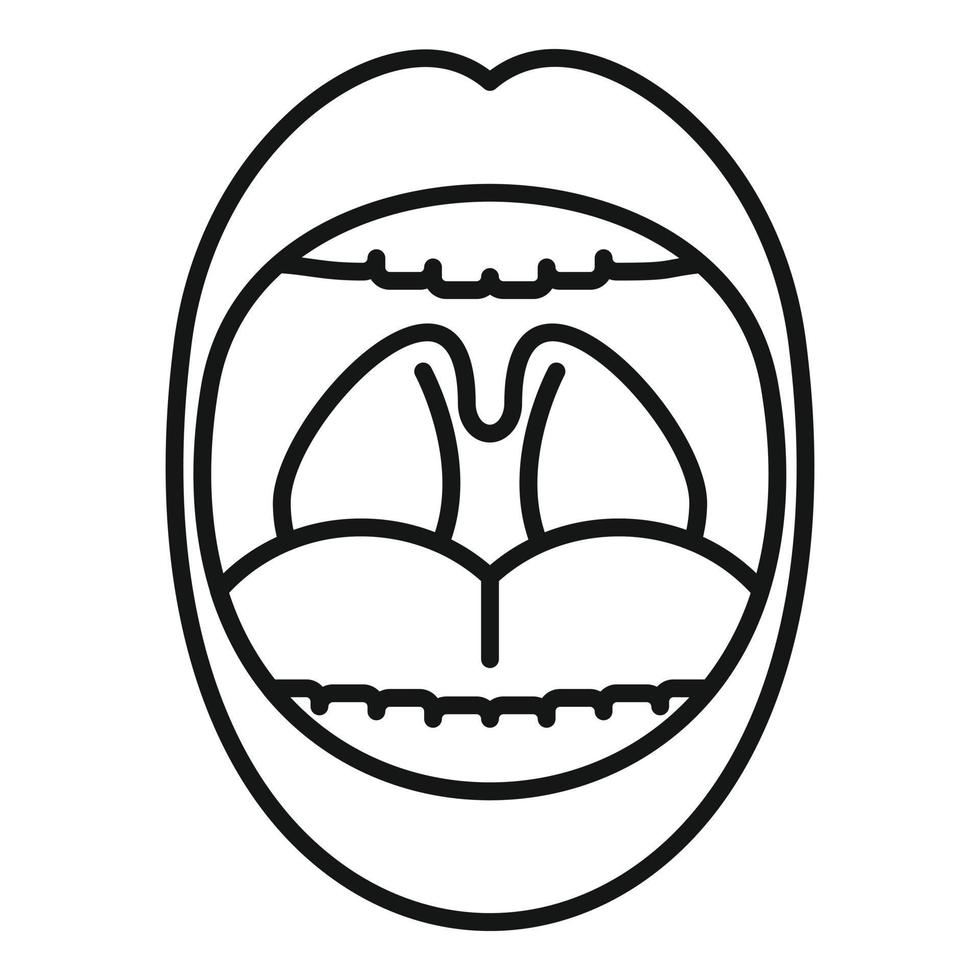The image is a stark, black and white, digitally-rendered graphic of an open mouth set against a pure white background. The exterior border of the mouth is an oval shape that tapers into a point at the top. Within this outer oval is another oval that forms the inner lip's border, emphasizing the open mouth's structure. Inside the mouth, you can see the top and bottom rows of teeth, the tongue, the uvula, and the gums on the sides. The artwork meticulously displays all the internal features of the mouth, including the striking detail of the back of the throat, accentuating the features like the tonsils and the roof of the mouth. The image excludes any additional background elements, maintaining a focus solely on the detailed and precise depiction of the mouth.